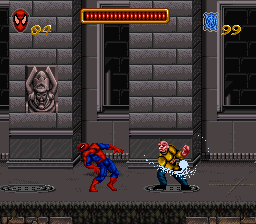This detailed image appears to be a small, illustrated screenshot from the Spider-Man game on the Sega Genesis, originating from either a screen grab or an emulation. The image depicts a battle between Spider-Man and a villainous henchman. Spider-Man, positioned to the left, is depicted mid-combat, appearing to be losing as he slightly falls back from a recent hit by his foe, who is on the right and standing on a manhole cover. The scene unfolds on a gray sidewalk in front of a large gray block wall that resembles a castle, complete with a gargoyle fountain head or a frightening creature with upraised hands set in stone. The façade includes a plaque featuring Galactus in the background, adding a cool Easter egg to the scene. In the upper left corner, there is a Spider-Man face logo displaying “04,” likely indicating Spider-Man's remaining lives. Beside it, a blue shield logo shows “99,” signifying the amount of web fluid available. A gold-edged rectangle bar runs across the middle of the screen, though its exact purpose is uncertain.